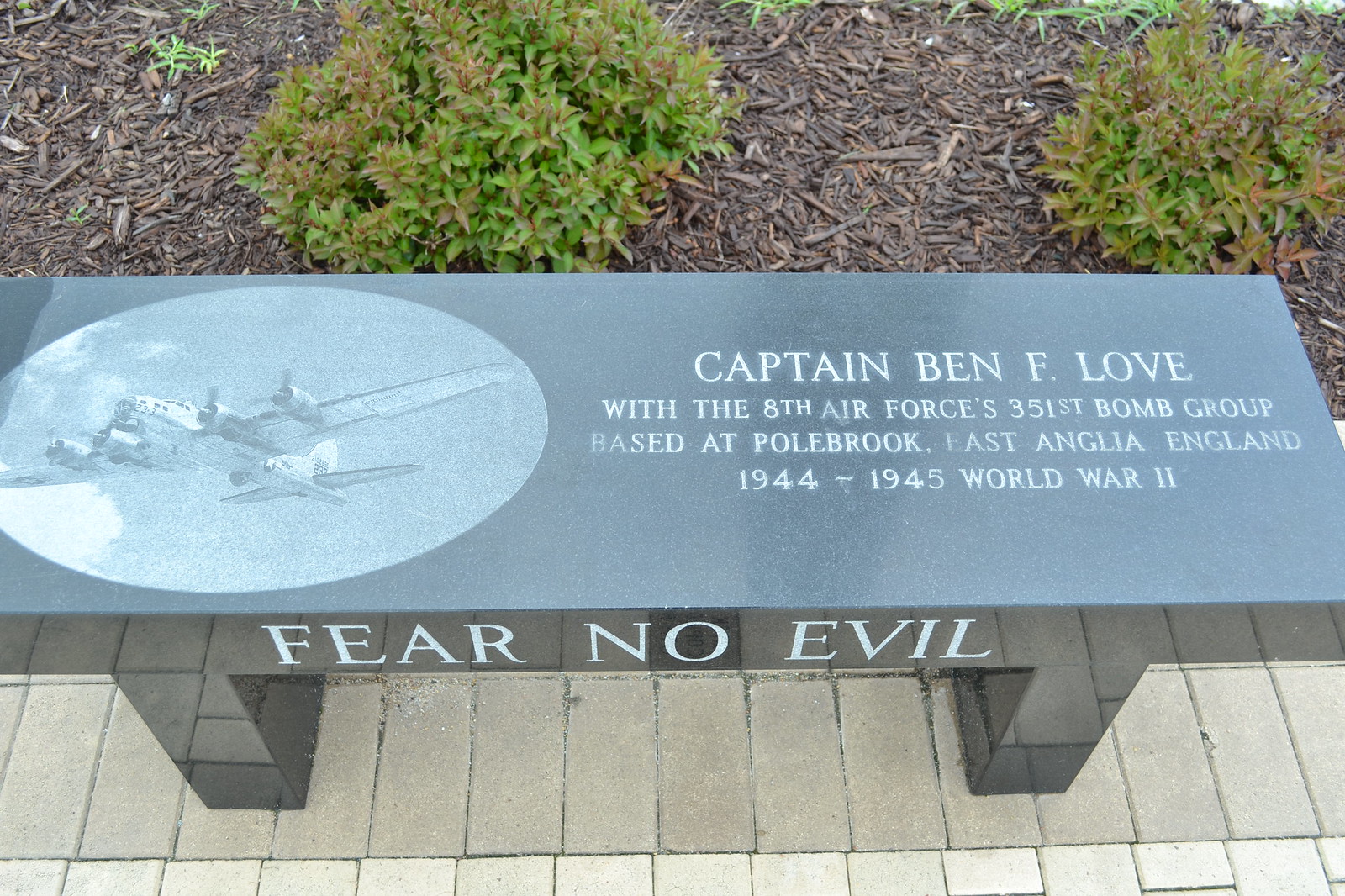A meticulously crafted bench made from dark gray granite honors Captain Ben F. Love of the 8th Air Force's 351st Bomb Group, stationed at Polbrook, East Anglia, England from 1944 to 1945 during World War II. Intricately inscribed in white on the right side of the bench, his name and military service stand as a testament to his bravery. The left side features an oval emblem with a detailed depiction of a white, four-engine bomber aircraft flying leftward, showcasing its expansive front wings and shorter rear wings. The front of the bench boldly displays the phrase "Fear No Evil." Positioned atop a bed of yellow-toned bricks, the bench is surrounded by a thoughtfully landscaped area featuring dark mulch and two verdant green bushes, interspersed with green leaves, some tinged with brown.